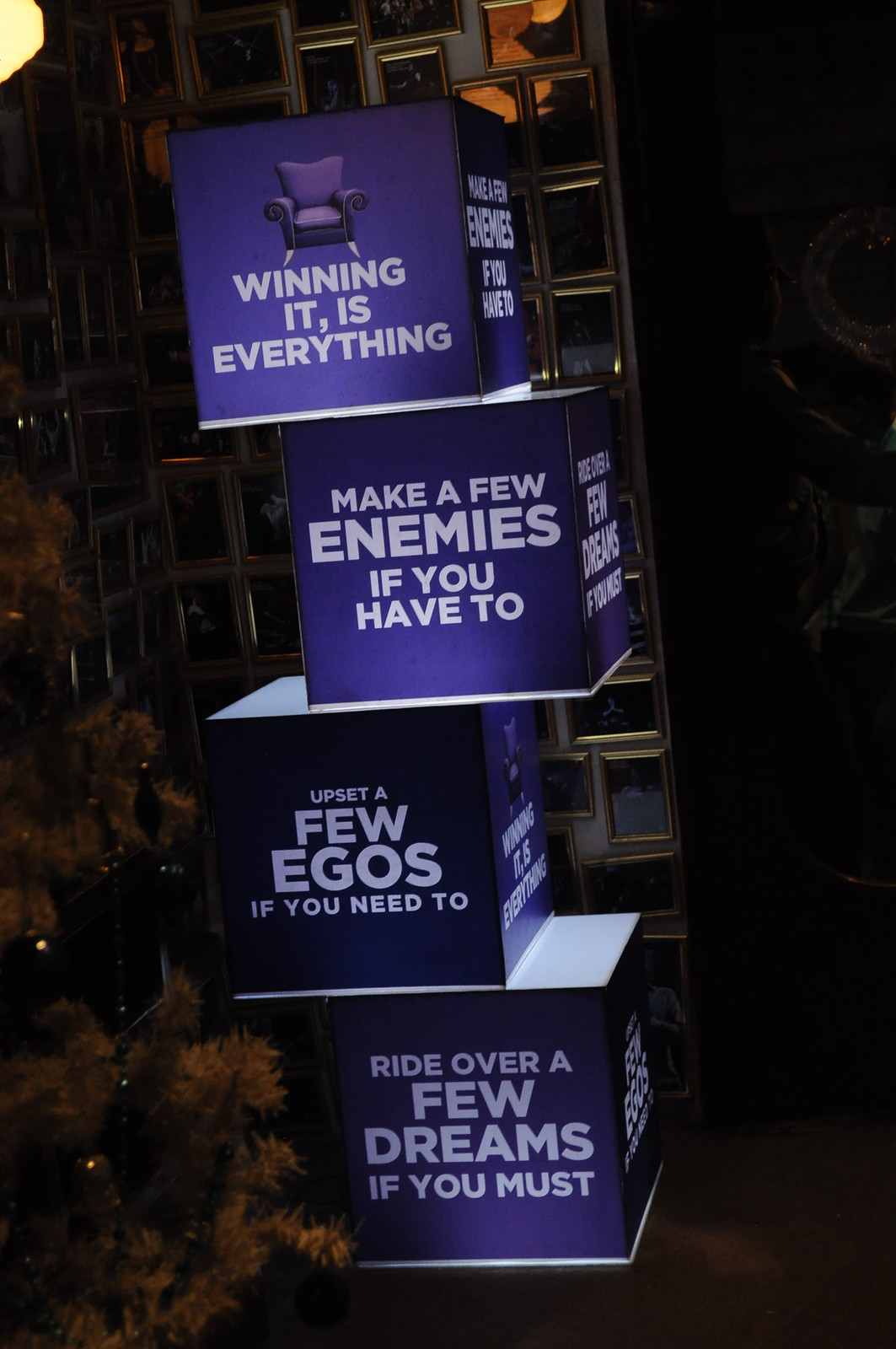The image depicts an outdoor scene with yellowish-brown leaves on the side and a shadowy, indistinguishable background to the right. Dominating the foreground is a stack of four purple and white three-dimensional boxes, arranged one atop another. Each box features bold white capital lettering. The top box, adorned with an image of a purple chair, bears the phrase "Winning it is everything." Just below, the second box, slightly askew, reads "Make a few enemies if you have to." The third box, also askew, states "Upset a few egos if you need to." The fourth and bottom box, resting on the ground, declares "Ride over a few dreams if you must." There's an additional presence of brown and black colors, though the dominant hues remain purple and white. Behind these boxes appears to be a wall with framed photographs, though the details are obscured. A hint of floral decoration is visible in the left corner, adding a touch of nature to the otherwise promotional setup, which is likely advertising something.